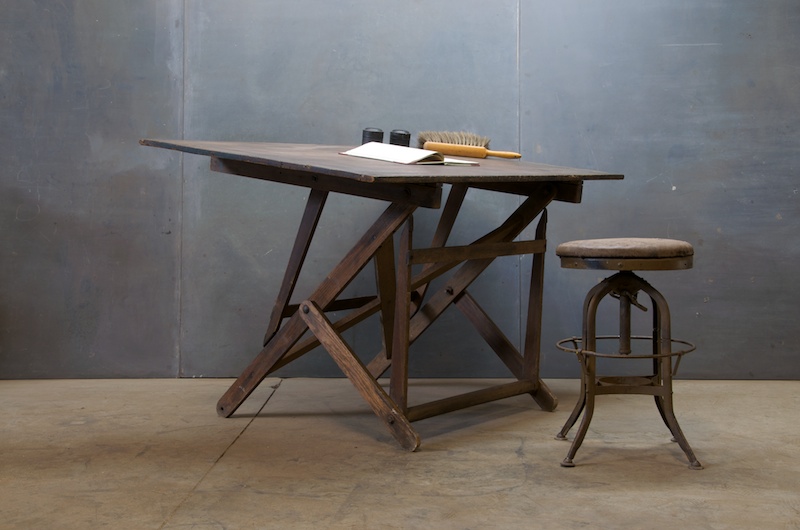The image is a detailed photograph of an antique drawing board and a stool, set against a plain gray wall with two visible seams. The drawing board, notably large and square, is tilted and rests on rudimentary, unpolished wooden legs. The intricacies suggest a possible mechanism allowing the desk to fold or tilt for ergonomic use. Accompanying the desk is a weathered stool to the right. This stool has a metal frame with a round, minimally padded seat, which appears dusty and old. Its base includes a tubular structure likely used for height adjustment. On the drawing board, there is an assortment of objects: a brush, two black containers that resemble salt and pepper shakers, and an open book. The floor beneath is tan with a noticeable seam running through it, adding to the overall antiquated ambiance of the room. There are no people in the scene, and it exudes a sense of historical utility and simplicity, focusing solely on the functional, yet aged furniture.